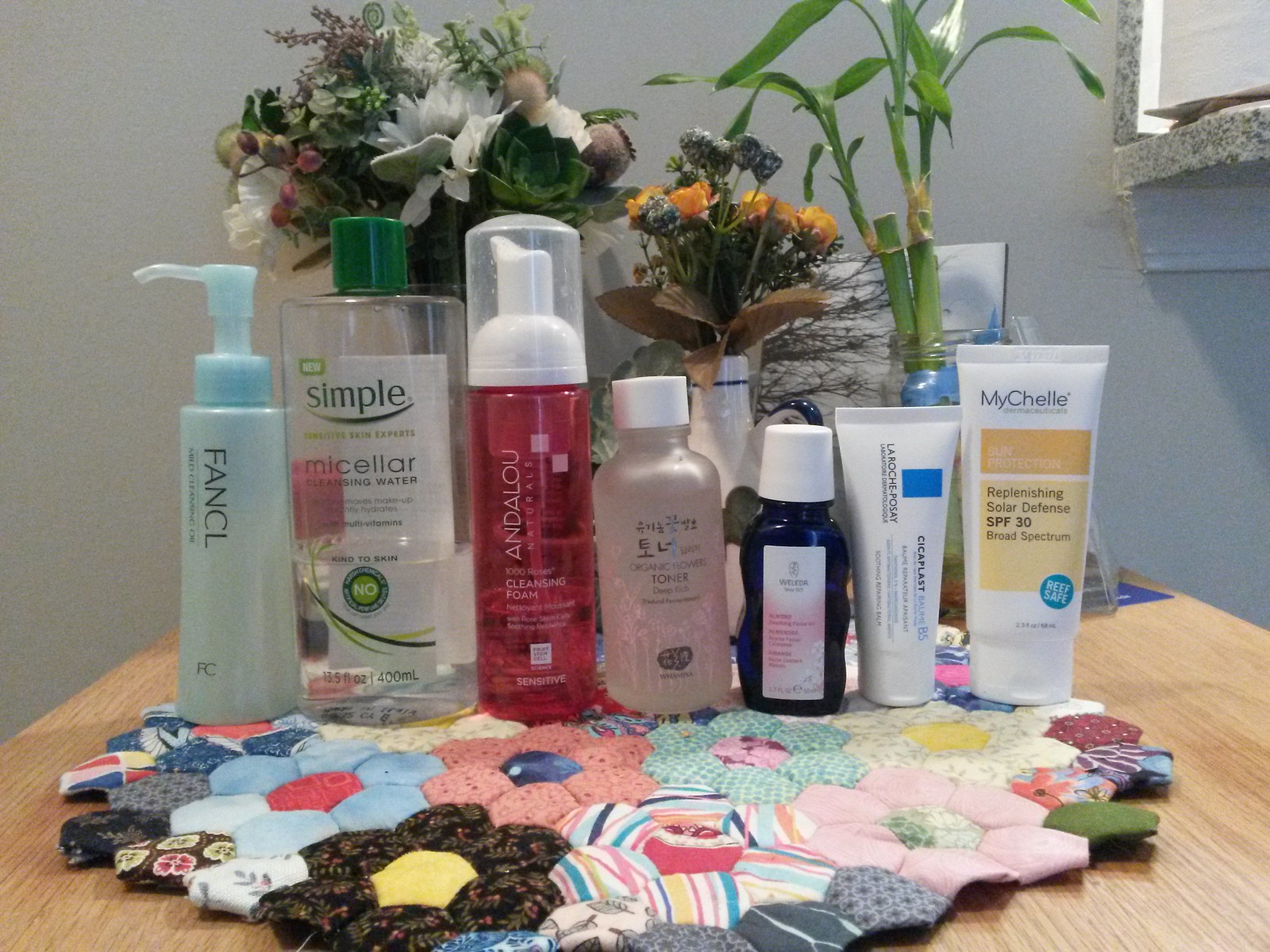The photograph captures a meticulously arranged product display in a corner of a beauty salon or spa, most likely aimed at enticing customers. The setup is on a wooden table positioned to the left of a granite countertop. This strategic placement ensures the display catches the eye of anyone passing by.

The focal point of the display is a circular, quilted mat composed of hexagon-shaped tufts, giving it a honeycomb-like appearance. Upon this mat, various beauty products are showcased, neatly arranged to highlight their brands and uses.

From left to right, the products include:

1. A **light blue pump bottle of Fancil**, its purpose unknown.
2. A **clear plastic bottle of Cleansing Water** by Simple, with a distinctive green cap.
3. An **aerosol foaming cleanser by Andalou**, in a vibrant red bottle with a pump top.
4. An **elegant, semi-transparent bottle** with a pearl sheen and a white top, its brand and function unspecified.
5. A **small navy blue bottle** paired with a white top.
6. Two upright-standing tubes of potential **face cream or facial liquid**, both utilizing the cap as their base for vertical display.
7. A **MyChelle replenishing Solar Defense SPF 30**, clearly labeled as such.

In the background, three vases filled with flowers add an inviting and aesthetic touch, enhancing the overall appeal of the display. This thoughtfully curated arrangement is clearly designed to attract customers and promote the sale of these diverse beauty products.